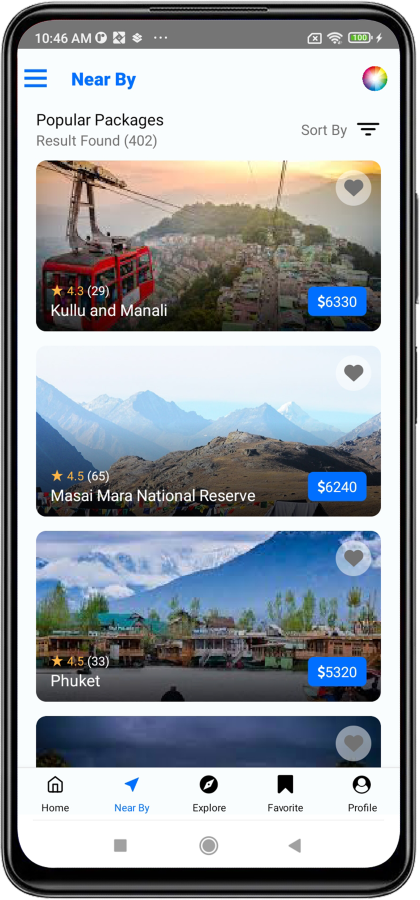The image displays a cell phone screen showcasing various travel packages. In the upper left corner, the time reads 10:46 a.m., and the battery indicator shows nearly 100% in green. Below this, there are three blue horizontal lines next to the word "Nearby."

Following this, the section titled "Popular Packages" appears. It lists 402 results and features an image of a cart heading down a mountain, with a rating of 4.3 stars. The location is specified as Kullu and Manali. The price is highlighted inside a blue rectangle as $6,330.

Another package listed is for Mesa Mera National Reserve, rated 4.5 stars, with an image depicting tall mountain peaks. The package price is $6,240.

Lastly, a package for Phuket, Thailand is featured, showing an image of numerous small houses or hotels set against a backdrop of a large blue and white snow-capped mountain. This trip is priced at $5,320.

The screen essentially highlights different popular travel packages available for booking.